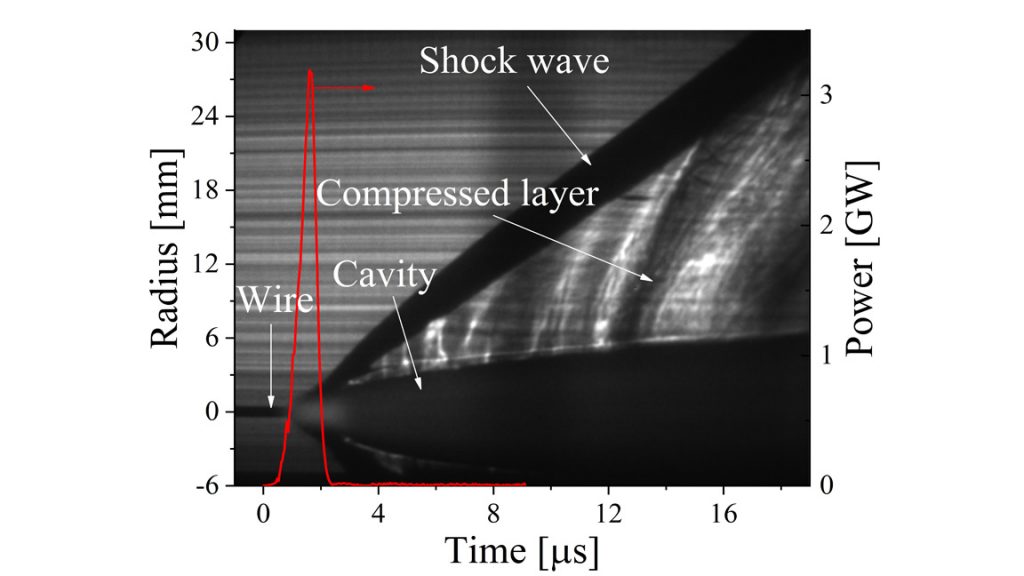The image depicts a detailed black and white graph titled "Exploding Electrical Wires Underwater to Understand Shock." The left vertical axis is labeled "Radius (mm)" ranging from -6 to 30, while the bottom horizontal axis is labeled "Time (μs)" ranging from 0 to 16. The right vertical axis is labeled "Power (GW)" from 0 to 3. The graph itself features several key elements: a black-to-gray gradient area illustrating different layers—including a black area denoting the compressed layer and a light gray area indicating a cavity. White arrows within the graph point to significant features labeled "Wire," "Cavity," "Compressed Layer," and "Shock Wave." A sharp, thin red line extends vertically from 0 to 30 on the left side and curves between 0 and 4 on the time axis, highlighting a significant radius measurement. The imagery suggests a scientific analysis of an exploding wire, possibly to study shock waves created underwater.